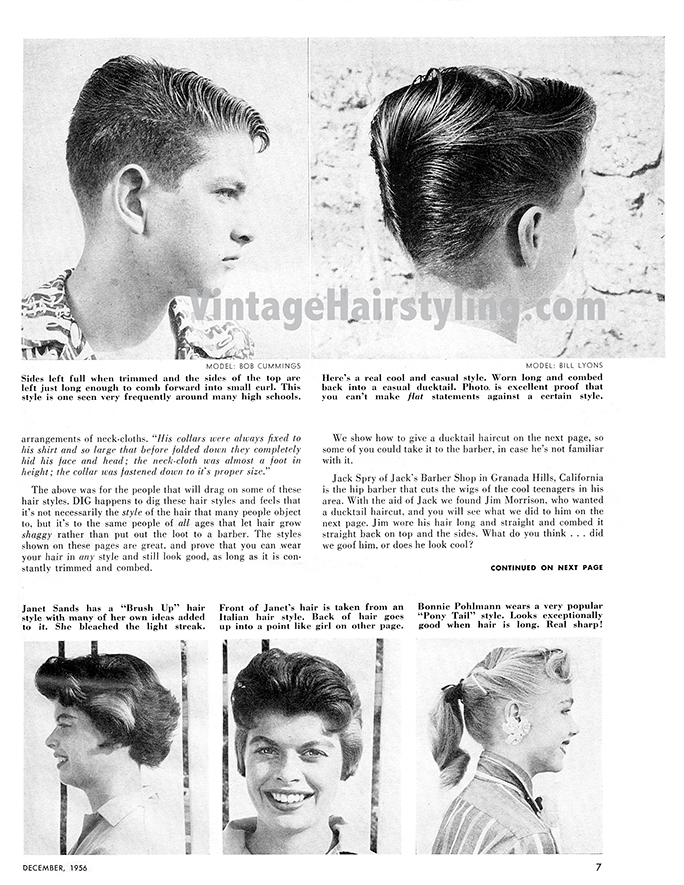The image appears to be a page from a vintage hairstyling magazine, dated December 1954, and sourced from the website vintagehairstyling.com. This black-and-white image features an assortment of period hairstyles. At the top, there's a young boy, possibly a tween or young teen, shown in two views: a right profile revealing short cropped sides and a longer greased forelock, and a rear view displaying a slicked-back, greaser style. Below, on the bottom half of the page, three black-and-white photographs depict women's hairstyles from the 1950s. The first two pictures show Janet, who has a short haircut styled from her left profile and head-on, featuring a bleached light streak in front, inspired by an Italian hairstyle, with the back styled into a point. The third image is of Bonnie, who resembles Olivia Newton-John’s character from "Grease," with blonde hair, curled bangs, and a curled ponytail. Each hairstyle reflects the popular trends of the 1950s, showcased in a magazine page exhibiting the era's iconic fashion.